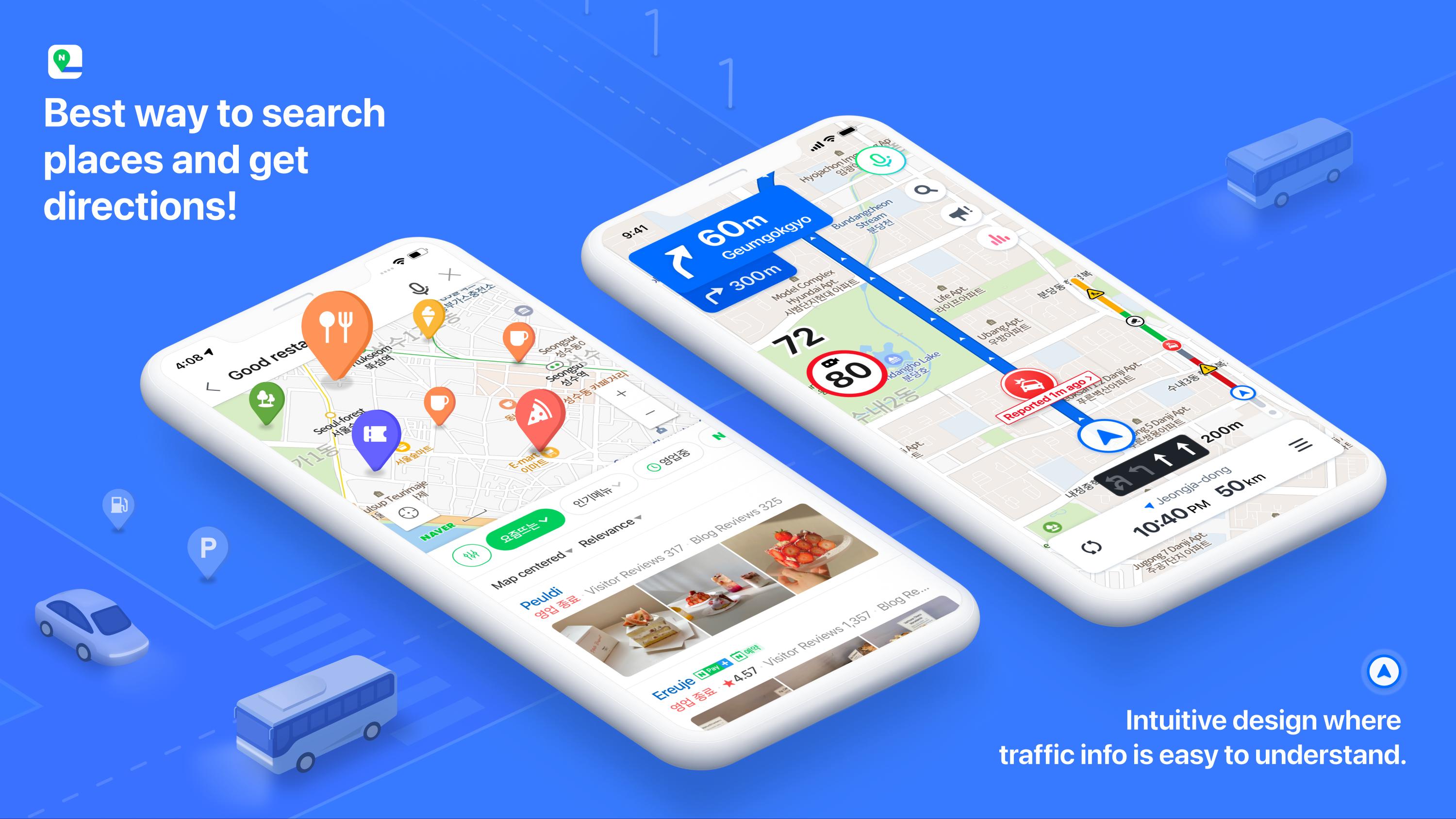This image features a detailed illustration on a blue background that appears to represent a digital map or navigation-related advertisement, possibly for a service like Hotels.com or Booking.com. The background displays a network of roads populated with cars and buses. Prominently featured is a white square containing a pin with an "H" (presumably indicating a hotel) accompanied by the text, "Best way to search places and get directions." 

The image includes various elements indicating additional functionalities:
- A gas pump icon and a parking pin, signifying essential travel amenities.
- Two mobile phones lying flat next to each other, each showing different types of information. 

The phone on the left:
- Displays various icons representing pizza, coffee, ice cream, food, movie tickets, and parks/recreation.
- It advertises "good restaurants" and features icons for a microphone and an "X," indicating a voice search function.
- It shows "408" and indicates location services are on, connected to Wi-Fi, with a half-full battery.
- The screen displays a list of restaurants, including "Paludi" with 317 visitor reviews and 325 blog reviews, and "Irizu" with 4.5 stars from 1,357 visitor reviews. Illustrations of strawberry cake are seen as examples of dishes.

The phone on the right:
- Displays navigation information, showing "60 miles to Grimgokyo" and directions to turn in 300 meters.
- Highlights recent updates stating an accident reported one minute ago, similar to Waze or Google Maps functionality.
- Shows a speed limit of 80 with corresponding signage, and a traffic camera icon.
- Lists details including "Zhangjidong, 1040 p.m., 50 kilometers," and various functional icons like a microphone, search, megaphone, and bar graph.

At the bottom of the image, a headline reads, "Intuitive design where traffic info is easy to understand," within a white circle edged in blue. This illustration underscores the image's focus on accessibility and ease of navigation features for users.